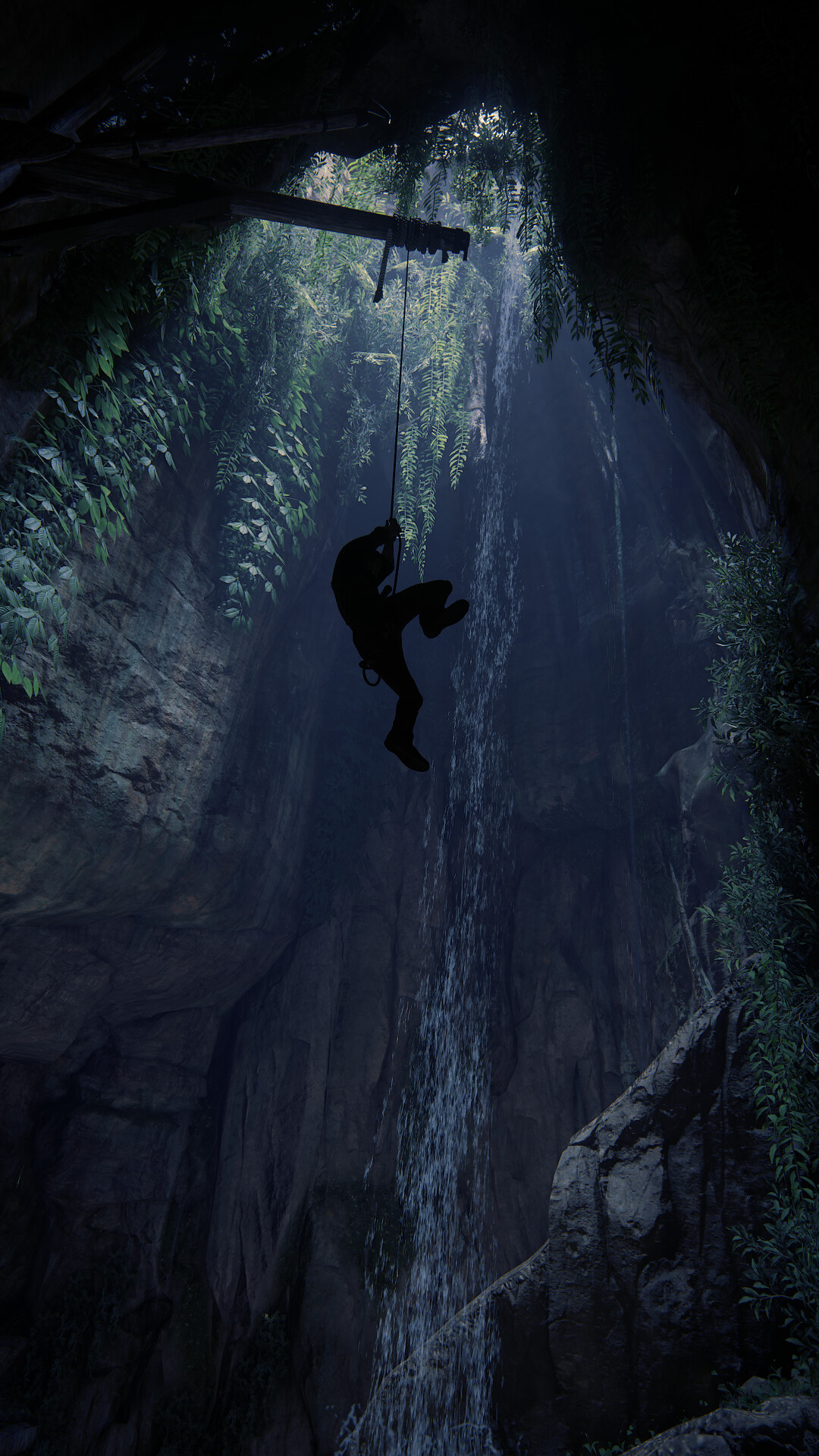In this compelling nature photograph, a person is dramatically captured in silhouette as they descend via a rope into a deep, dark cave. The silhouette of the individual, positioned roughly halfway down the image, highlights their adventure into this natural wonder. Above, a small opening allows slivers of sunlight to filter through, faintly illuminating the cavernous space. This light source reveals stunning natural rock formations that frame the scene and support patches of greenery and vines clinging to the rugged walls. Further enhancing the ethereal atmosphere, a waterfall cascades gracefully from the top, its source obscured by the shadows. The scene is viewed from below, gazing upwards towards the bright, foliage-fringed entrance, making the silhouette and the surrounding environment appear even more dramatic and awe-inspiring.